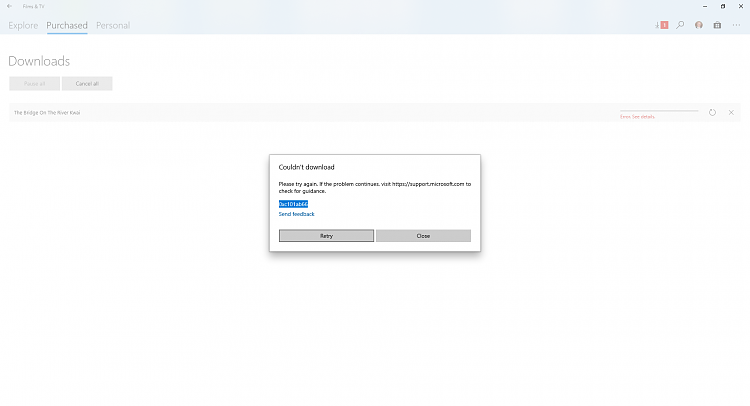This image depicts a web application interface designed for films and TV shows. The interface appears to be displayed on a desktop, as indicated by the window controls (minimize, maximize, and close) located at the top right corner of the screen. 

At the top of the web app, there are three main tabs labeled "Explore," "Purchase," and "Personal." The "Purchase" tab is currently selected, as evidenced by a blue underline beneath it.

On the far right side of the interface, four smaller icons are arranged vertically. These icons include, from top to bottom, a business or home icon, a magnifying glass for search purposes, a user profile icon, and a shopping bag icon, likely for cart or purchase-related functions.

Below the main navigation tabs, there is an error message displayed within a white rectangular notification. The message reads: "Couldn't download. Please try again. If the problem continues, visit https://support.microsoft.com to check for guides." Adjacent to this error message, some code snippets are also visible.

The overall theme and structure of the web app suggest a well-organized platform, with a focus on user navigation and functionality for purchasing and exploring film and TV content.